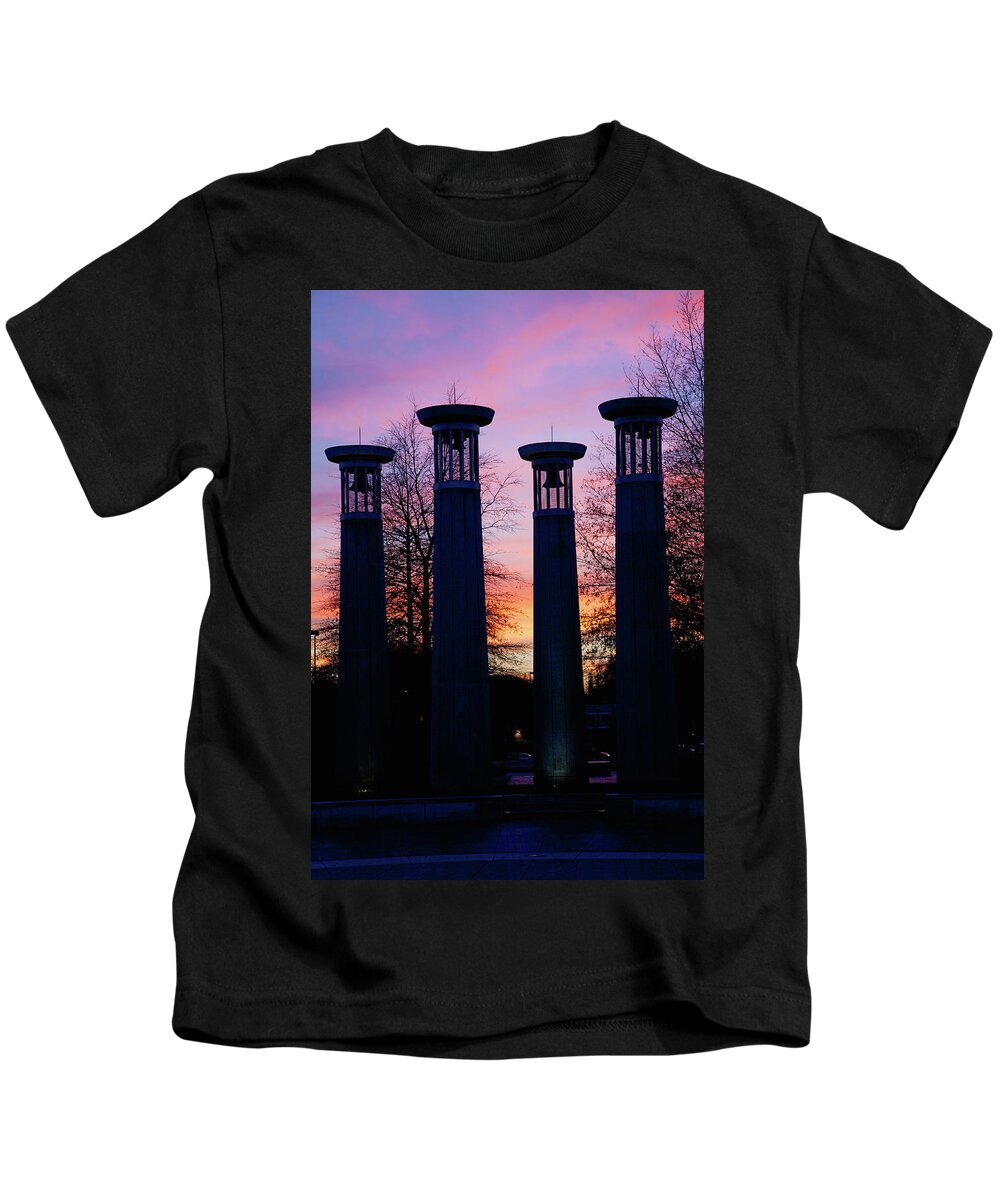The image depicts a black t-shirt laid on a white background, with a printed photograph prominently displayed on the shirt's front. The photograph, appearing digitally imposed due to the absence of shirt wrinkles, captures four short bell towers silhouetted against a vibrant dusky sky. The atmosphere suggests sunset, as the sky transitions from vivid oranges at the horizon to softer pinks, purples, and blues higher up. The towers, each housing visible bells through their mesh windows, stand in stark shadow, with details obscured due to the evening light. Surrounding the towers are bare, silhouetted trees, adding to the serene yet somewhat mysterious ambiance. Below the towers, vague outlines hint at a wall and a possible walkway, suggesting the scene might be in or near a park setting.